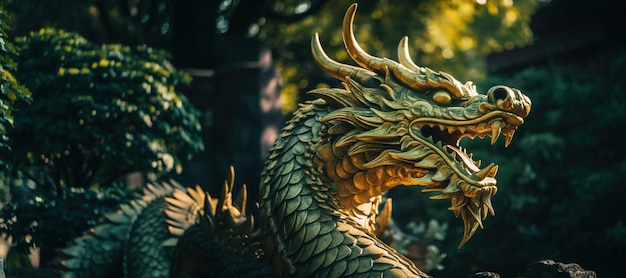The image captures a highly realistic and detailed statue of an Oriental-style dragon, predominantly featuring its menacing head. The dragon’s head, adorned with intricate golden scales under its chin and metallic green across its body, displays sharp teeth emerging from an open mouth, ready to attack. Its eyes are a striking bead-like gold with no visible pupils, enhancing its fierce appearance. The dragon's body, decorated with spikes and spires, coils behind it, adding to its dynamic pose. The statue, which appears to be set outdoors, is bathed in sunlight that highlights its glossy, metallic paint, giving it an almost lifelike sheen. The background is a blurred mix of green bushes, various shrubs, and trees, with some areas illuminated by sunlight, suggesting the setting might be a garden or park. The overall composition is rectangular, with the dragon facing to the right, making it a captivating focal point against the subdued, natural backdrop.